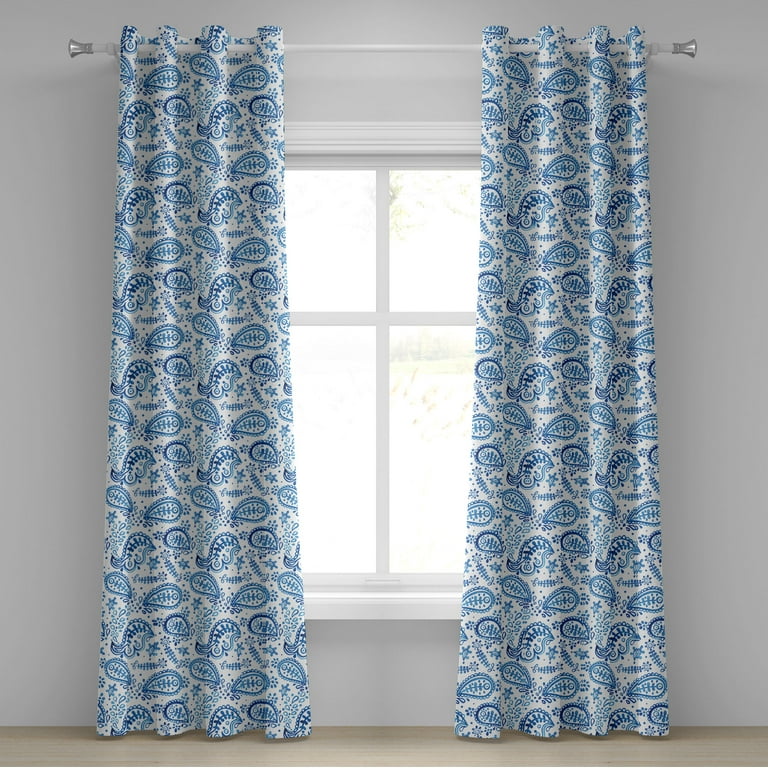The image depicts a vertical rectangular window in a room with light gray walls and a bare, light brown wooden floor. The window, framed in white and consisting of two wide panes, is closed but illuminated with light filtering through. It is adorned with an elegantly white curtain rod, mounted about a foot above the window with round silver-colored end caps. Hanging from the rod are two pleated curtains, each featuring an intricate blue pattern against a white background. These curtains, parted in the center to reveal the window, extend from the rod all the way to the floor. The blue design on the curtains includes ferns and abstract shapes, creating a visually captivating contrast against the soft gray wall. Through the window, a lush green lawn can be faintly seen outside.